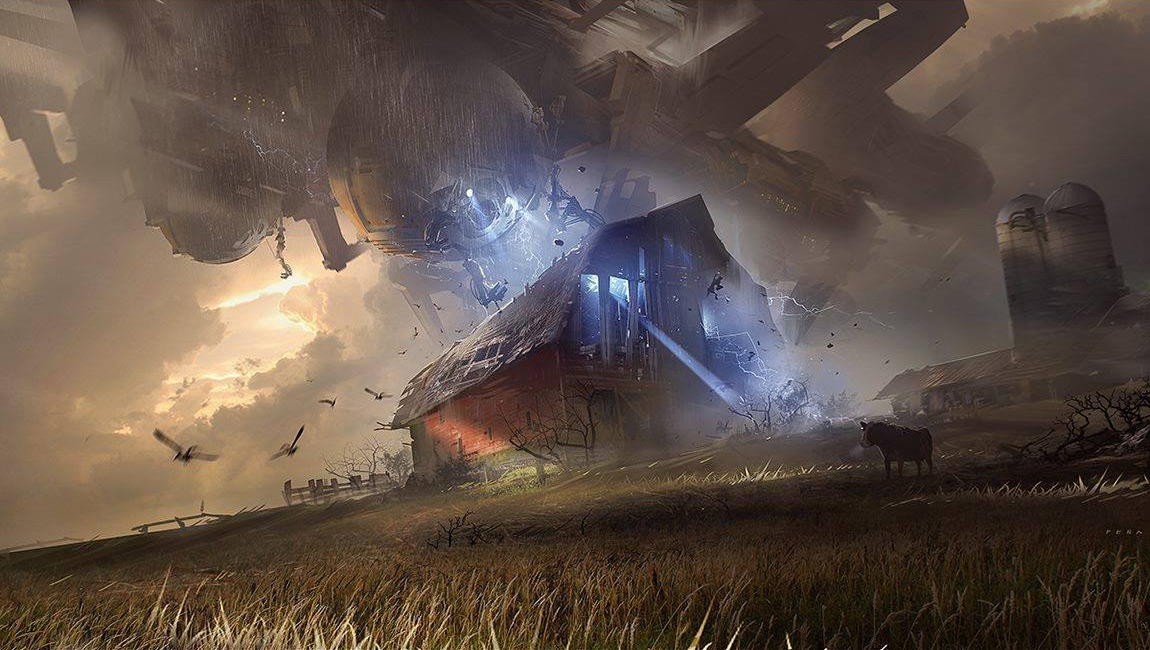In a stunning and evocative sci-fi concept illustration by Eduardo Pina, we witness the dramatic scene of an alien invasion. The image, rendered from a ground-level perspective, shows a red farmhouse in a brown hay or wheat field at center frame. Silhouetted against the chaotic backdrop are gray shadowy silos and building structures to the right of the barn. As a colossal alien spaceship, with a dome-like front emitting twin rays of light, hovers menacingly close to the buildings, the barn is violently dismantled. Its walls explode outward, the roof splits asunder, and debris is flung into the air. Adding to the turmoil, crows scatter in all directions, disturbed by the invasion. Deep, dark clouds dominate the sky, illuminated by a sliver of intense sunlight breaking through on the left. In the pasture on the right, cows stand unfazed amidst the destruction, providing a stark contrast to the extraterrestrial chaos unfolding above.